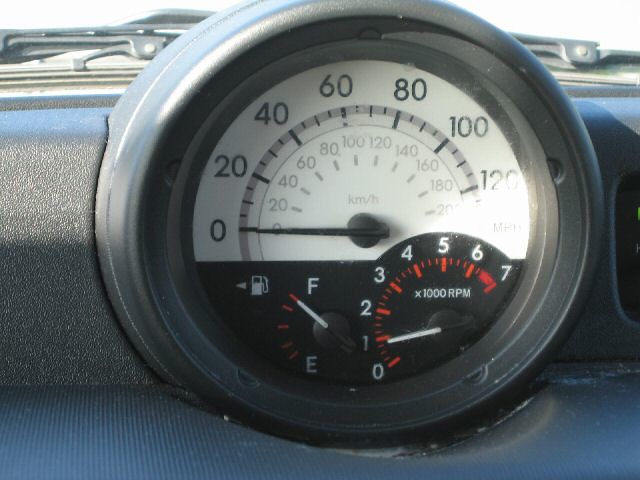The image depicts a car's dashboard, specifically focusing on the speedometer, which is encased in a gray plastic frame. Surrounding this frame, glimpses of the car's body and windshield wiper are visible, along with the windshield itself. The speedometer display ranges from 0 to over 120 mph, with black numerals and dashes marking each increment. Below this, there is a smaller scale showing kilometers per hour, ranging from 0 to over 200 km/h, displayed in a gray font.

Additionally, the dashboard includes a fuel gauge to the left of the speedometer. The gauge features a gas tank icon, with an "E" (empty) at the bottom and an "F" (full) at the top. Currently, a small white needle is pointing towards the "F," indicating a full tank. To the right of the fuel gauge, there is an RPM (revolutions per minute) meter that reads "x1000 rpm," ranging from 0 to 7. The numerals on the RPM meter are in white, while the small markers are in red. Currently, the RPM needle is positioned at 1, meaning the engine is idling at 1,000 rpm.